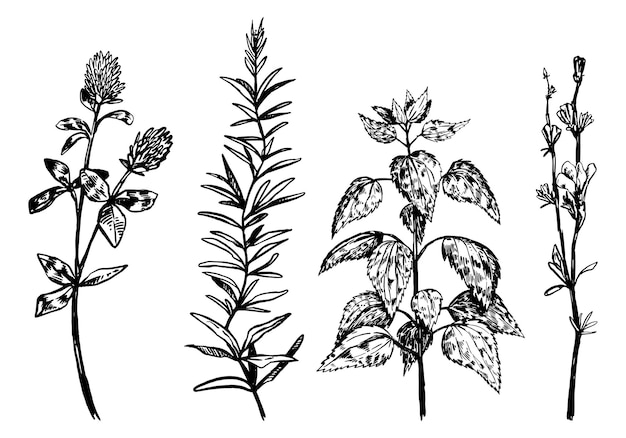The image is a detailed, black and white hand-drawn sketch of four different plants against a plain white background, possibly from an illustration in a book. Starting from the left, the first plant features a thin stem with several leaves extending from the sides and two flowers blooming at the top. The second plant, taller and skinnier than the first, has numerous thin leaves running along its height but no flowers. The third plant exhibits large, heart-shaped leaves that hang down from the stem, with the leaves decreasing in size toward the top. The rightmost plant is the spindliest, with a thin stalk that splits halfway up. This plant has fewer, long and thin leaves, with a small flower halfway up one of the splits and more leaves near the top.